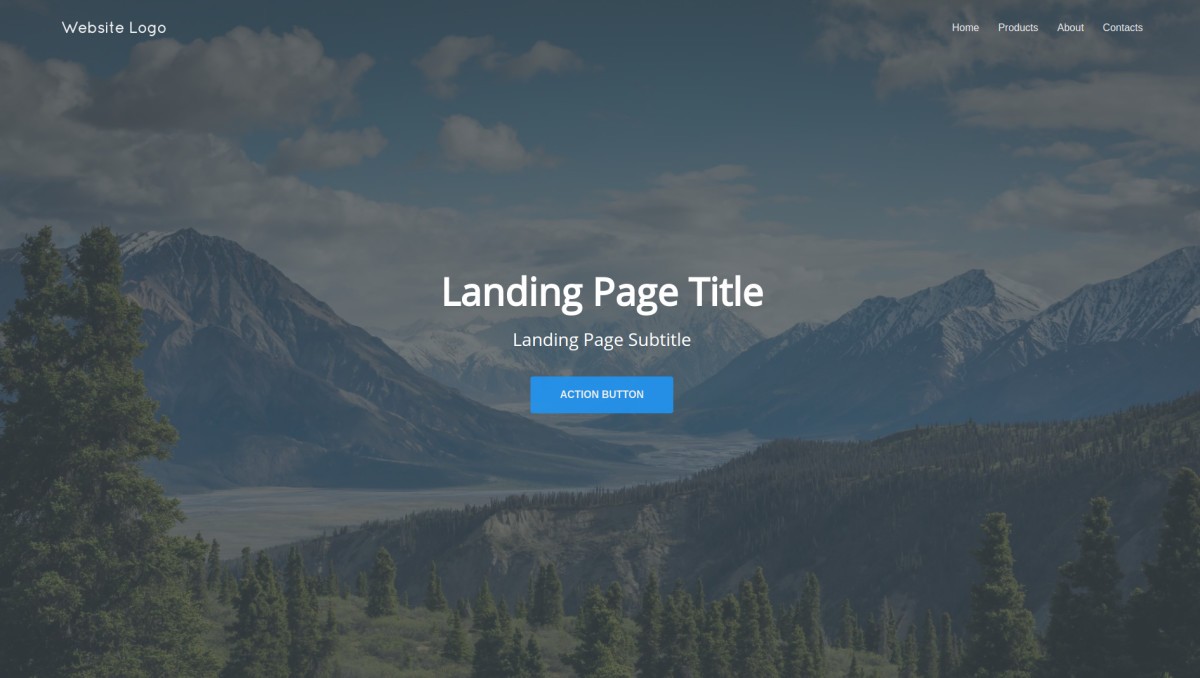This image showcases a picturesque landscape featuring majestic mountain ranges in the background, with a serene lake or river meandering between the peaks. The lush greenery, dotted with beautiful trees, enhances the natural beauty of the scene. The sky is a brilliant blue, punctuated by scattered clouds, indicating a bright, sunny day.

Superimposed on this scenic backdrop is a template for a website landing page. At the top of the page, there are prominent white letters that read “Landing Page Title,” “Landing Page Subtitle,” and an “Action Button.” In the upper left corner, the text “Website Logo” is displayed in white. Along the right side of the image, there is a navigation menu with options for “Home,” “Products,” “About,” and “Contacts.”

The sleek and clean design of this landing page template makes it an excellent choice for anyone seeking a visually appealing and user-friendly website framework. The blue action button stands out against the scenic background, guiding the user to take the next step. This template is both aesthetically pleasing and practical, allowing users to easily customize the title, subtitle, and action button text to meet their specific needs.